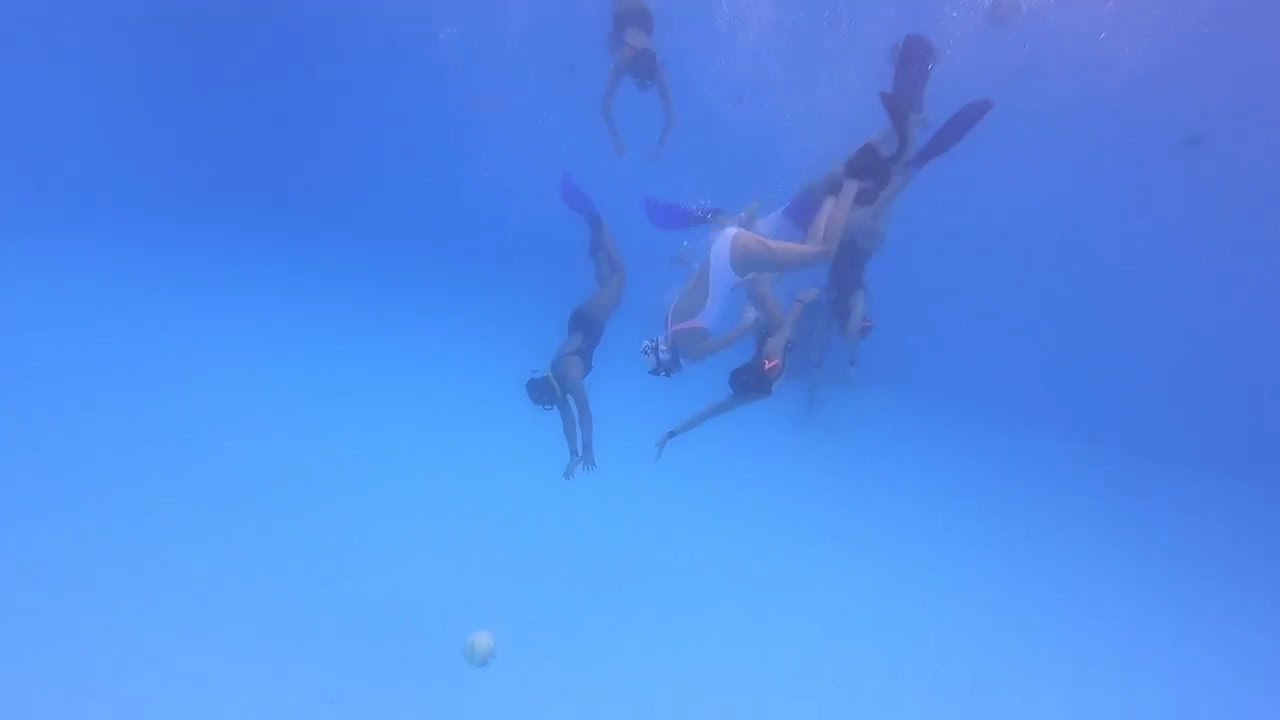Beneath the ocean's surface, in a slightly blurry but vibrant scene of light and dark blue waters, five women are swimming downward towards a white ball resting at the ocean floor. The swimmers, all equipped with goggles and fin flippers for better movement, are dressed predominantly in black webbed swimsuits, except for the central figure who stands out in a white swimsuit and matching swim cap. The top portion of the ocean appears darker blue, contrasting with the lighter blue of the lower part where the women are actively swimming. The sense of depth and movement is palpable as they converge towards the ball, creating a dynamic and captivating underwater moment.